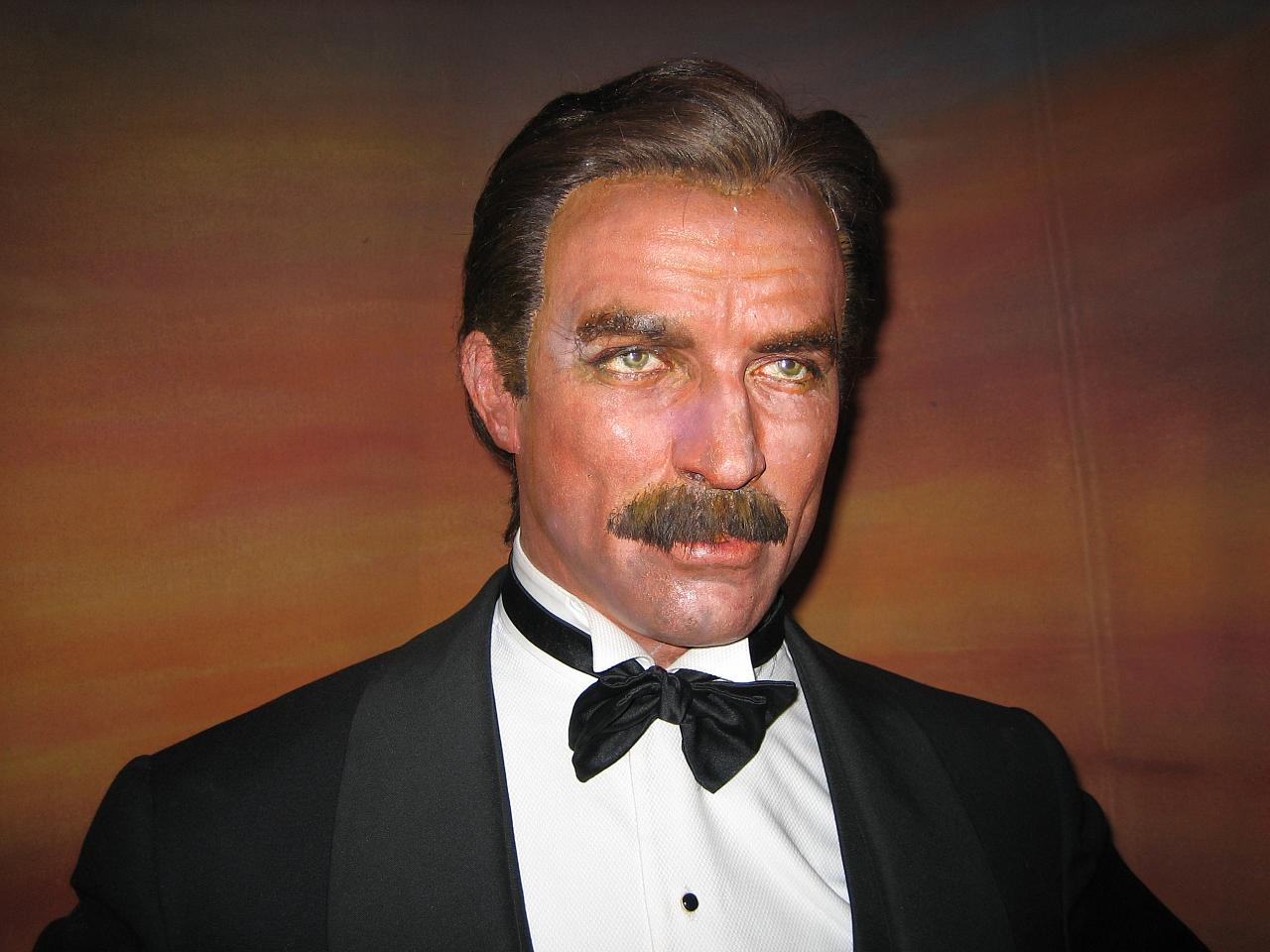The image features a lifelike wax figure of a white male resembling Tom Selleck, known for his dark, slicked-back brown hair and iconic bushy mustache. The figure is dressed in a black tuxedo jacket with lighter black on the collar, a white high-collared shirt adorned with black buttons, and a black bow tie. His green eyes, thick brown eyebrows, and detailed facial texture reflect the meticulous makeup used to create his likeness, giving him a somewhat serious expression with a hint of a smile. The background is a painted mural with hues of orange, brown, and yellow, evoking a sunset or skyline with clouds sweeping across the scene. The overall composition, including the artificial hair and skin hues, maintains the illusion of realism, making the figure appear real from a distance.